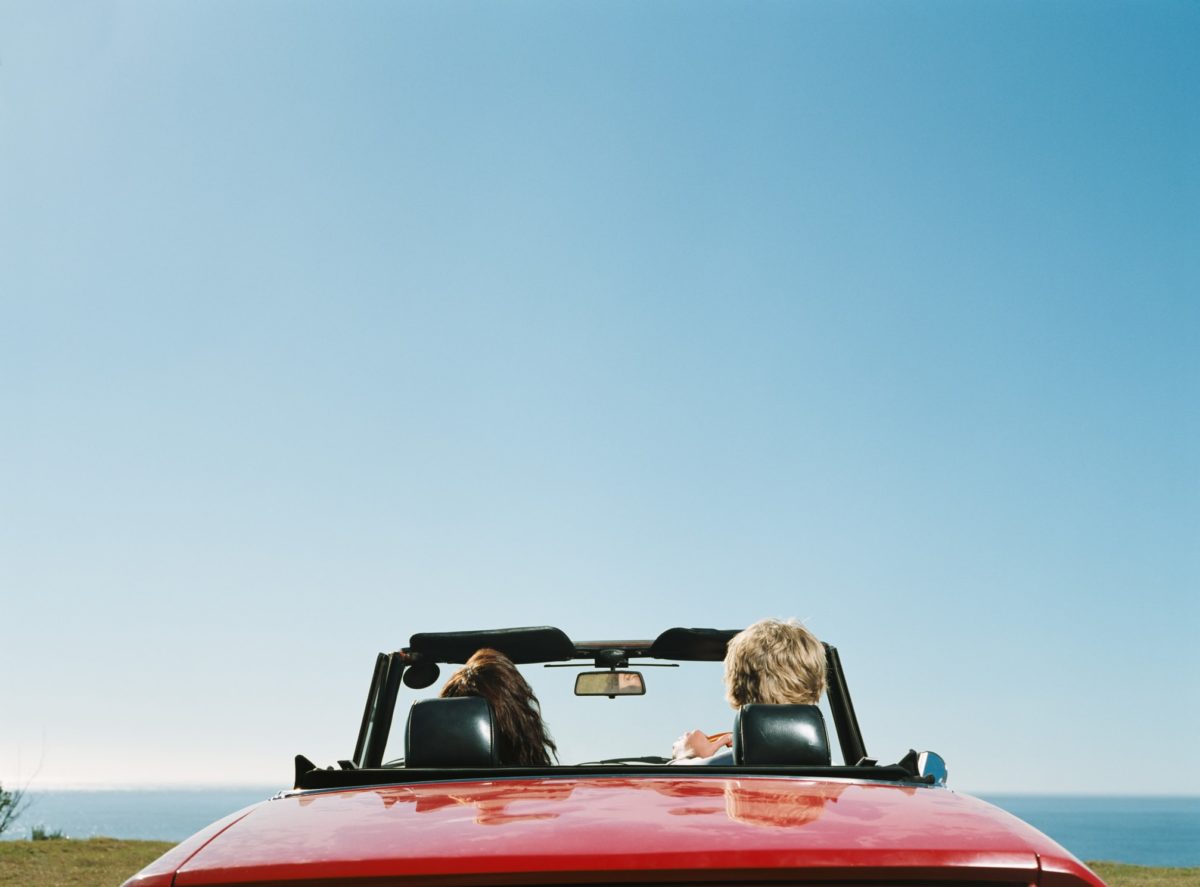In this photo, a couple, possibly a man with light blonde hair and a woman with dark brown hair, sit in a shiny red convertible parked at the edge of a cliff overlooking a hazy blue ocean. The image is captured from behind the vehicle, with the top down, revealing both occupants. The man is in the driver’s seat on the right, his hands on the steering wheel, while the woman is in the passenger seat on the left, her face partially visible in the rear-view mirror and her head resting against the headrest. The lower portion of the image shows a patch of green grass on either side of the car, indicating the cliffside setting. The couple gazes out in relaxed awe at the ocean, which stretches out before them, occupying the bottom half of the photo. The majority of the upper part of the image is dominated by the bright, clear, blue sky, creating a serene and expansive backdrop.